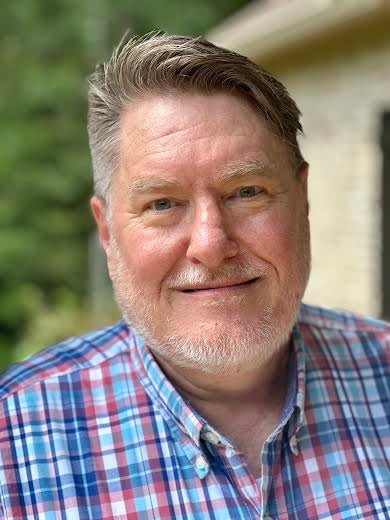This is a detailed close-up photograph of Les Ferguson, likely a biblical author, shot from the chest up. He is wearing a blue, red, and white plaid Oxford shirt, facing directly towards the camera with a small, thin smile. He appears to be in his late 60s, with short, graying brown hair combed to the left, and a thin beard that is mostly white and connects to a matching thin mustache. His eyes appear to be light brown or blue, and he has a Caucasian complexion. The background suggests an outdoor setting, with blurry greenery and a house on the right side, adding additional context to the scene.